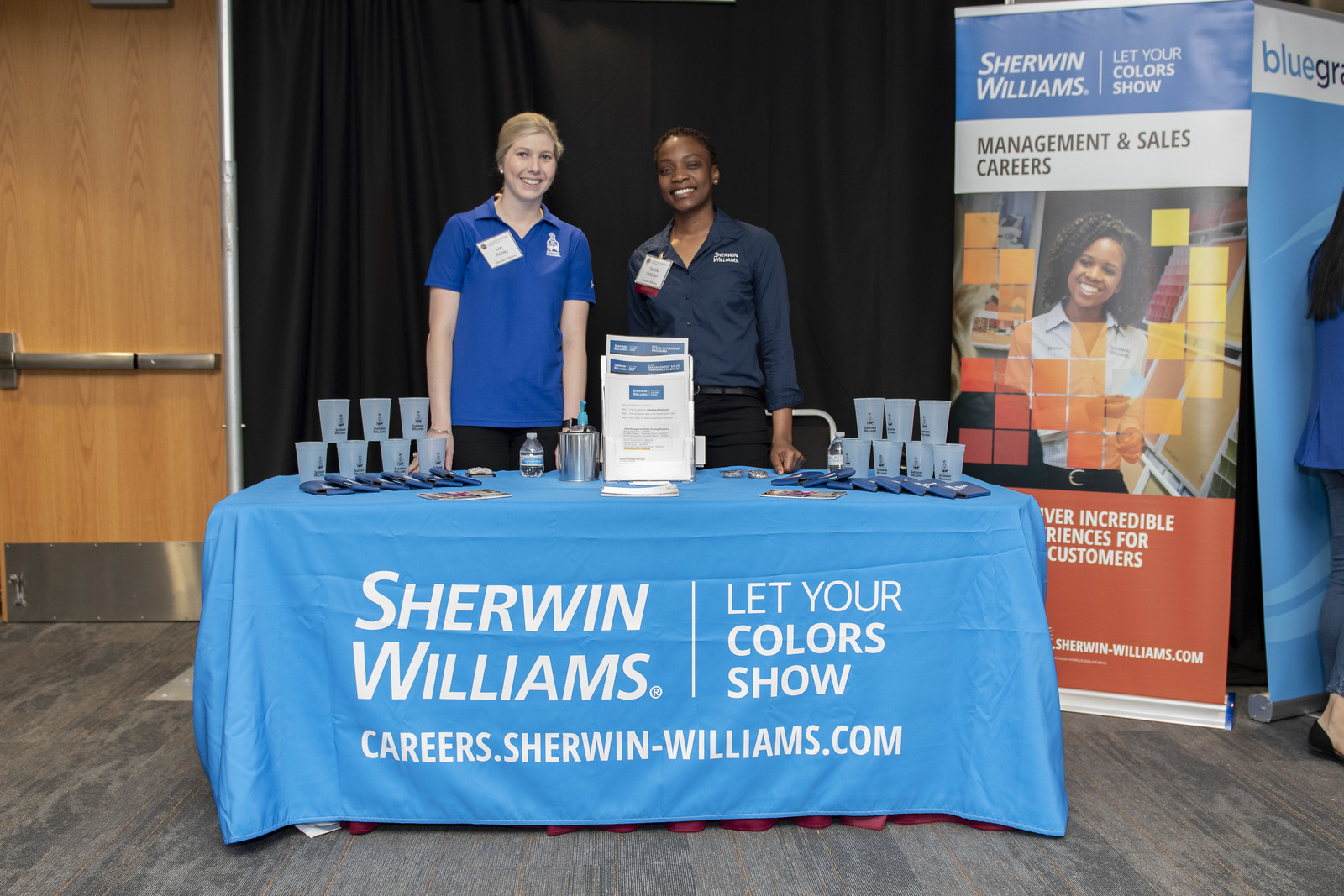This photograph captures a detailed scene at a Sherwin-Williams paint company booth, likely set up in an indoor expo center or trade show environment. Central to the image is a table draped with a blue tablecloth that prominently displays the Sherwin-Williams logo, the slogan "Let Your Color Show," and the website "careers.sherwinwilliams.com" in white text. The table is adorned with small promotional items such as cups, coasters, keychains, and informational flyers that outline career opportunities with the company. 

Behind the table stand two women, exuding a professional demeanor with welcoming smiles. The woman on the left is white, and the woman on the right is African American; both are dressed in blue shirts and have their hair neatly pulled back into ponytails. To the right of the table is a large boxy poster that reiterates the Sherwin-Williams branding, featuring text such as "Management and Sales Careers" and the slogan "Let Your Colors Show," along with partially visible phrases about providing incredible experiences for customers. 

The backdrop behind the women is a solid black, and to the left, there is a closed brown wooden door with a metal push handle. The overall environment is colored with various shades, including light blue, orange, yellow, brown, blue, black, tan, gray, white, beige, and silver, contributing to a vibrant and professional display at the trade show or expo center.